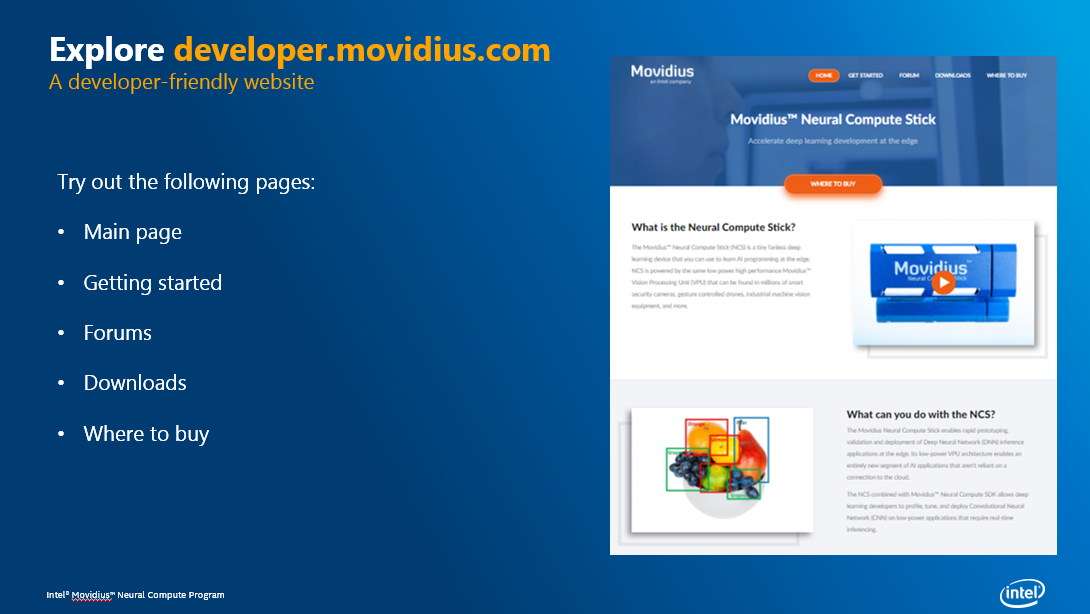The image features the homepage of the developer-friendly website exploredeveloper.movidius.com. The background transitions from a dark blue on the left to a lighter blue on the right. The title "Explore Developer" is prominently displayed in large white font, with "movidius.com, a developer-friendly website" written underneath in smaller orange font.

Below the main title, there is a section in white font advising users to "try out the following pages," followed by bullet points. The listed pages are: 

- Main page
- Getting started
- Forums
- Downloads
- Where to buy

Further down, in very small print, it says "Intel Modius" with "Modius" underlined with a red squiggly line, accompanied by the text "neural compute program."

On the right side of the image, several pages of the Modius website are partially visible, including the home page and a page titled "Modius Neural Compute Stick: accelerate deep learning development at the edge." Overlapping these is another page titled "Where to Buy," along with a heading that reads "What is a neural computer stick?" The content below this heading is in black font on a white background but is too small and low-resolution to read clearly.

Additionally, there is a video thumbnail featuring the text "This is Modius" with an orange circular play button that has a white arrow. Below the video, there is a heading reading "What can you do with NCS," with further text that is similarly unreadable due to poor resolution.